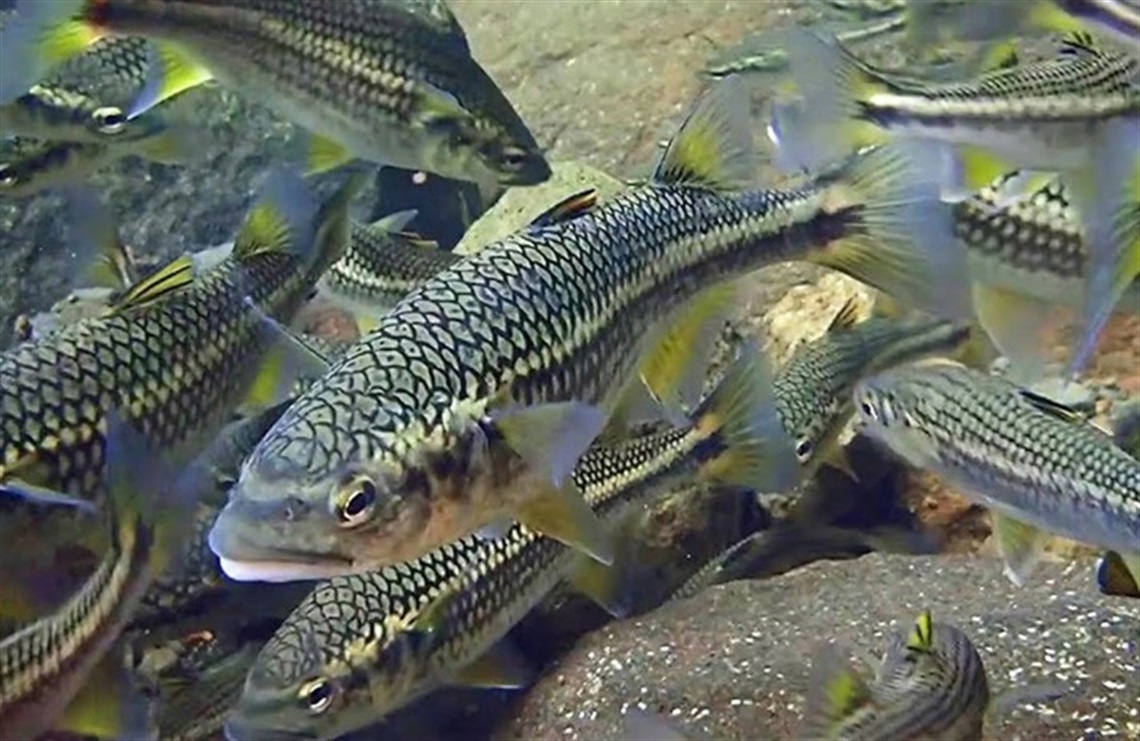This is an underwater photograph taken in a clear freshwater body, possibly a lake or a stream. The water is exceptionally clear, allowing a detailed view of the rocky bottom, which is scattered with stones. The key subjects are several fairly large fish, all of a similar species, populating the scene. The fish display shimmering greenish-yellow scales that transition to black, especially near their tails and fins. Their fins transition from black to yellow and then to almost transparent. Several fish are visible, with one prominent fish swimming diagonally across the center of the photo, moving to the left. You can see its eye and mouth clearly. Beneath this main fish, an identical one is closer to the bottom. Additional fish of the same kind swim in various directions, with some displaying full body profiles while others are seen from different angles, showing mostly their tails and top fins. The bright daylight reflects off the fish and rocks, enhancing the clarity and vividness of the underwater scene.